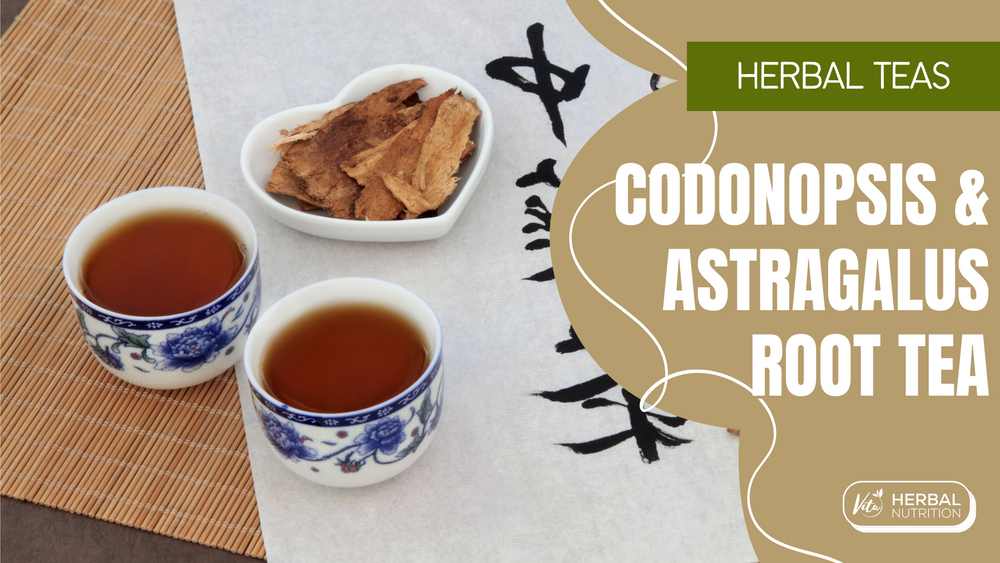This digital advertisement features an image on the left side showing two elegant white teacups adorned with blue floral and vine designs, filled with a rich brown tea. These cups are placed on different surfaces: one rests on a light brown bamboo table mat, visible at the bottom left corner, while the other sits atop a white fabric with black Chinese lettering. Nestled between the cups is a heart-shaped white dish containing a fibrous, brown and tan substance. The right side of the image showcases a green rectangular area with text detailing the product. In sleek white writing, it states "Herbal Teas," followed by "Codonopsis and Astragalus Root Tea" in capital letters. Additional text encircles the box with phrases like "herbal nutrition" and the brand "Vita Herbal Nutrition" towards the bottom. This visually appealing advertisement skillfully merges traditional tea time aesthetics with informative branding.